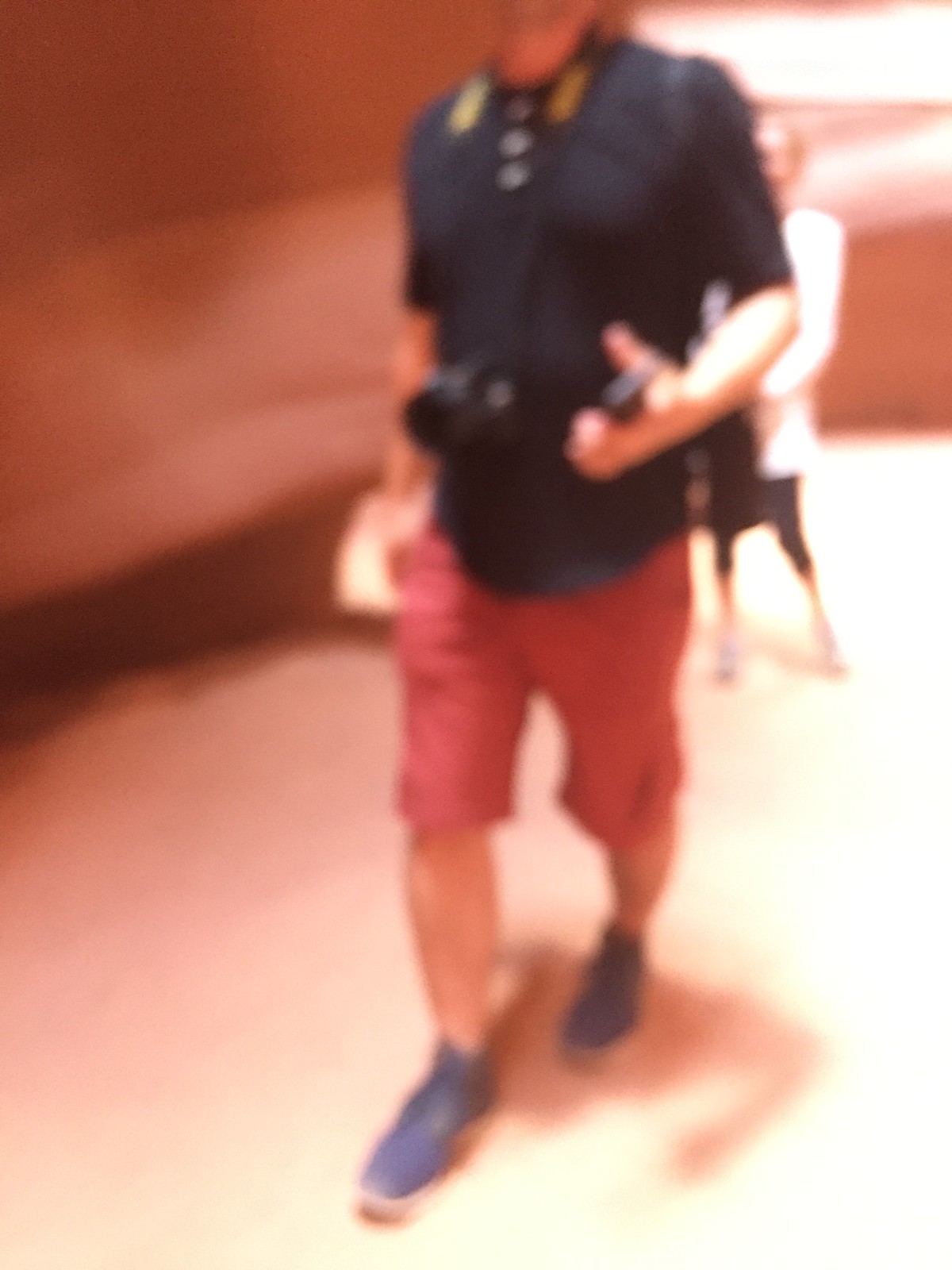In this blurry photograph, a man walks towards the camera, seemingly focused on something ahead. He is casually dressed in a short-sleeved black t-shirt, complemented by red shorts and blue sneakers. Around his neck hangs a camera, suggesting he might be a photography enthusiast. Notably, the collar of his t-shirt is accented with a yellow trim featuring three buttons. In his left hand, he appears to be holding a phone. The background of the image is dominated by a peach hue, possibly indicating a wall or building. Behind the man, a second figure is visible, likely a woman. She is dressed in a long-sleeved white shirt, black capri pants, and seems to be wearing sneakers as well, although her features are less distinct due to the photo's blur.